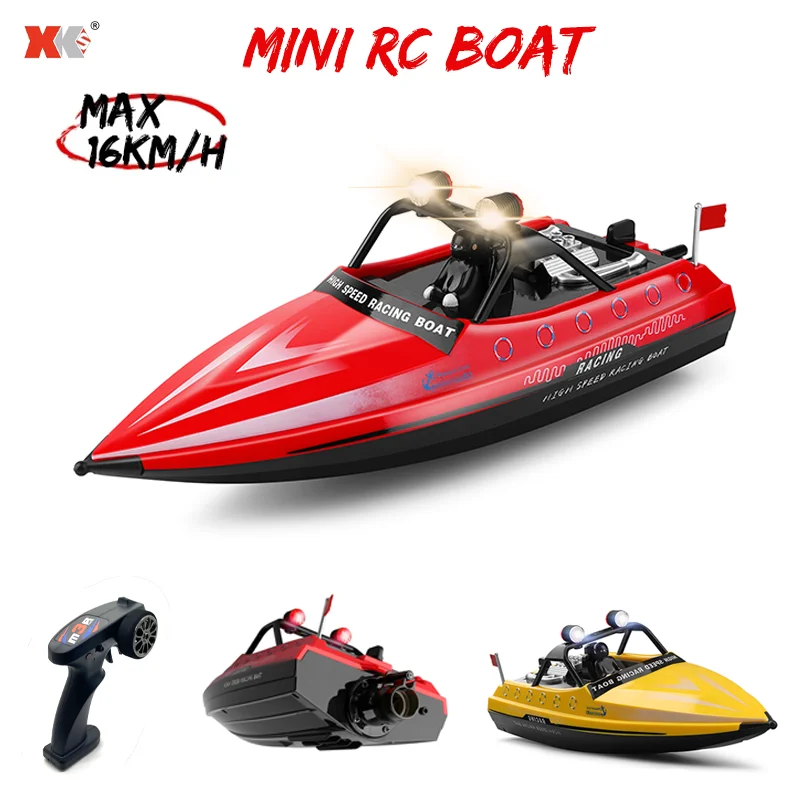This is an image featuring a Mini RC Boat prominently centered against a white background, with additional smaller photos below. The boat in the middle is a high-speed racing model with a red top and black bottom. It sports two glowing lights on its top and a small red flag at its rear. A plastic man, dressed in black with white hands, sits in the driver’s seat holding the steering wheel. Above the boat, bold red text reads "Mini RC Boat," and black text indicates a maximum speed of 16 kilometers per hour. The manufacturer's logo, "XKS," is in the top left corner.

Below the main image, there are two smaller pictures: the left one shows the back view of the red boat, highlighting a possible propulsion system, and the right one displays the same boat in yellow, with the text "Racing Speed Boat" visible but mirrored. To the far left of these smaller images is a photo of the remote control, featuring a single trigger and a tire-shaped steering wheel.